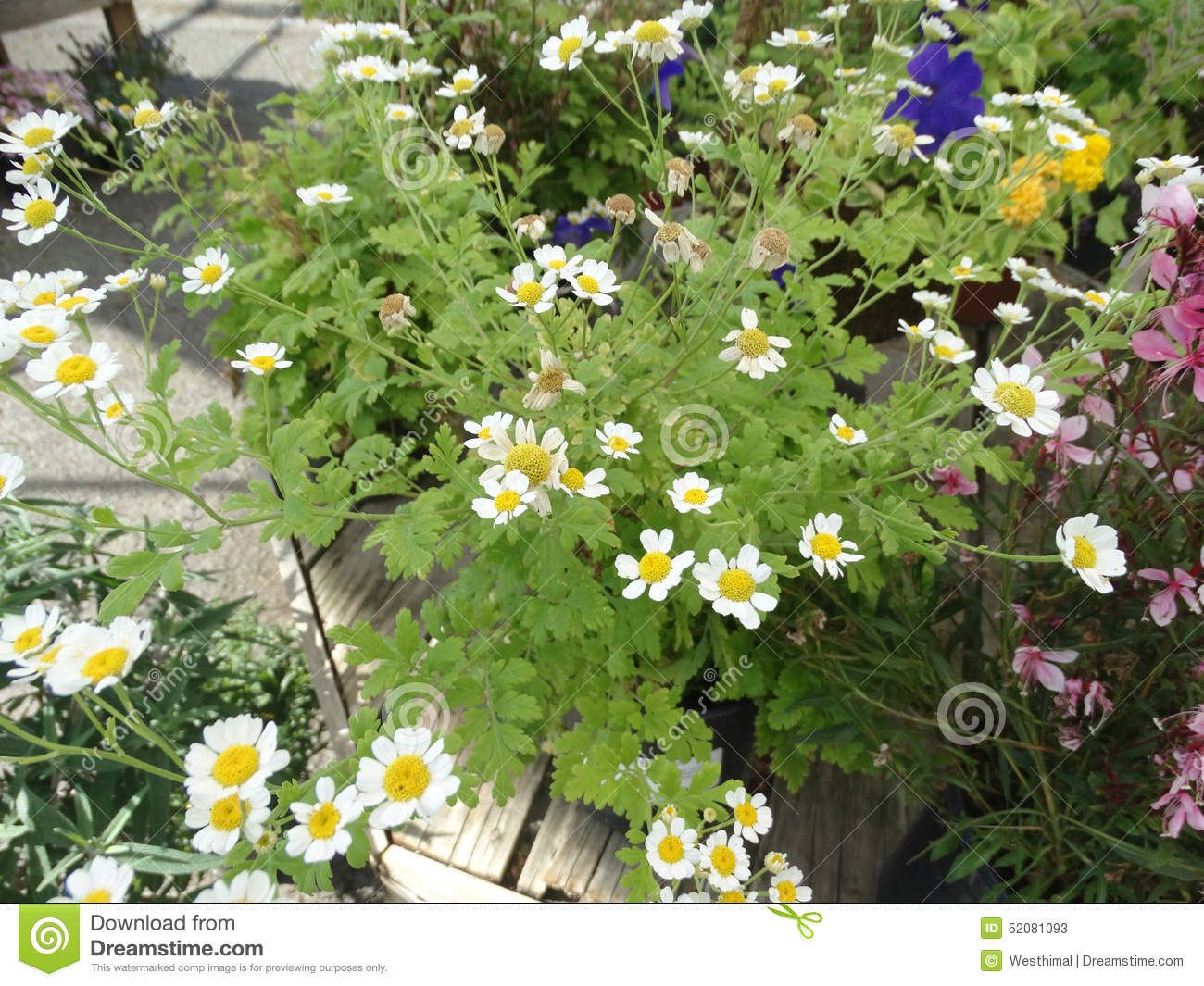A watermarked image from Dreamstime.com, ID 52081093, captured by westhimaldreamstime.com, shows an abundant growth of white wildflowers with yellow centers, characterized by numerous small white petals. These flowers, resembling daisies, are accompanied by green leaves that resemble cilantro, suggesting they are wildflowers flourishing freely. The image appears to feature these wild blooms around a wooden walkway, such as a patio or boardwalk. In the background, there is a presence of other colors, including dark pink and red flowers with pink leaves on the right side. Additionally, a swirl design and a scissors icon are visible in the composition. The background includes hints of blue hues and shadowed areas, providing depth and contrast to the vibrant flowers. This image, marked as a comp and available for previewing purposes only, is notable for the "Dreams Time" watermark and the associated copyright disclaimer.